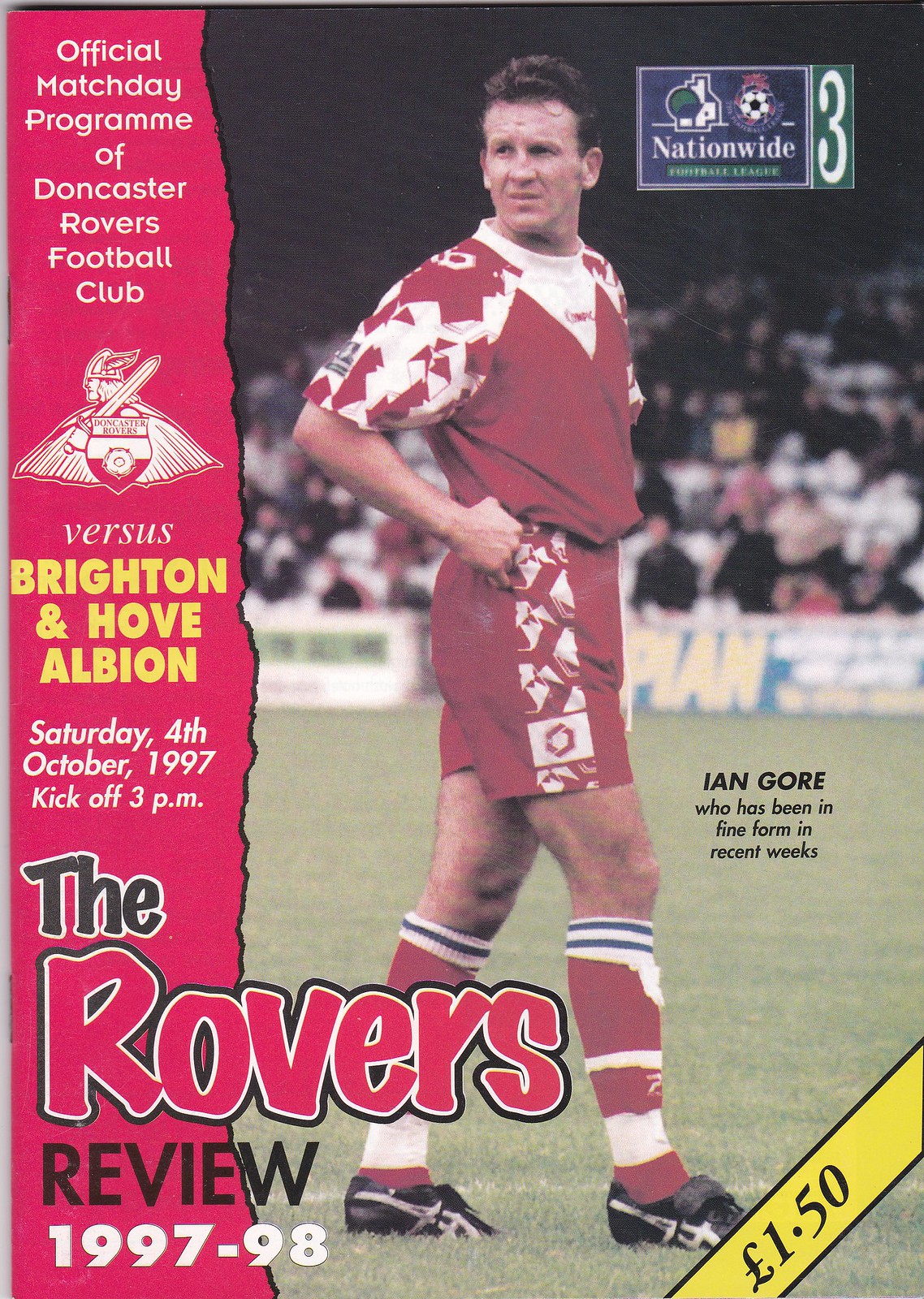This photograph, captured as a magazine cover, features Ian Gore, a soccer player in excellent form in recent weeks, sporting a red and white jersey, shorts, and socks, complemented by black sneakers. He stands with his hands on his hips, looking to the right, positioned on a grass field. The background is blurred, revealing a crowd of spectators in the stands. The left side of the cover is dominated by a red section containing the text: "Official Match Day Program of Doncaster Rovers Football Club vs. Brighton & Hove Albion, Saturday 4th October 1997, kickoff 3pm." Prominently displayed in large letters is "The Rovers Review 1997-1998." The lower right-hand corner lists the price, £1.50, while the top right corner features an advertising logo with a soccer ball and a house, indicative of the nationwide football league. Additionally, there’s an image of a Viking with a shield and sword, adding to the thematic elements of the cover.